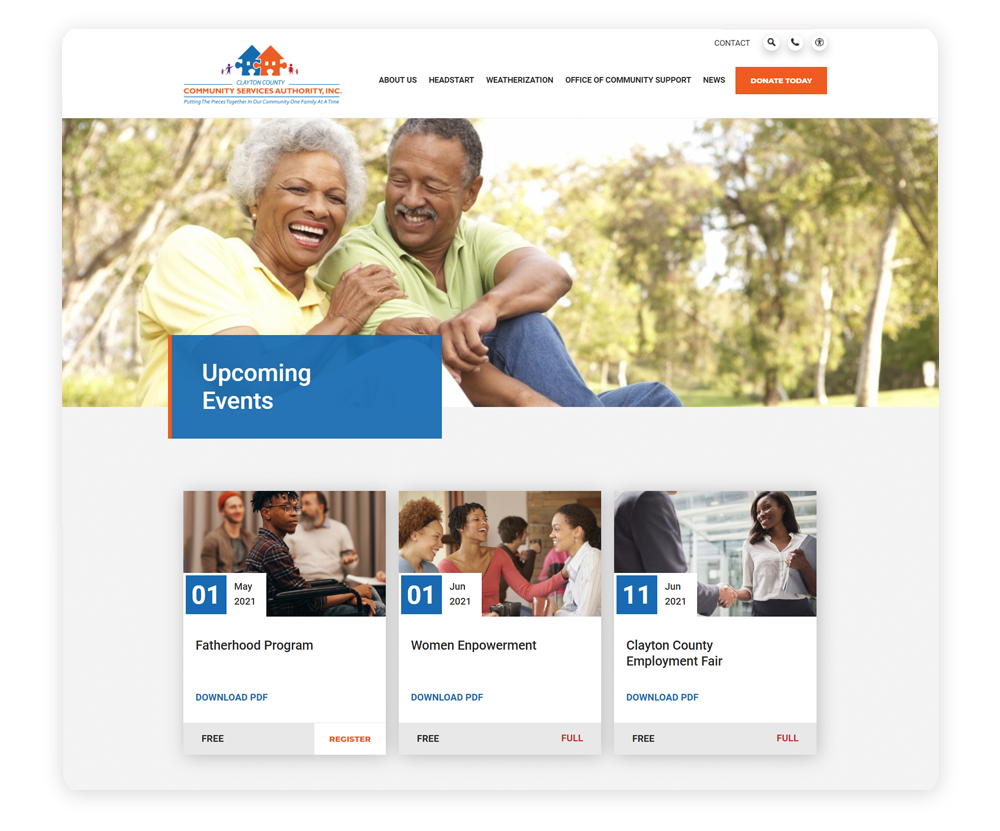Screenshot from the Clayton County Community Services Authority, Incorporated's webpage, showcasing the "Upcoming Events" section. The webpage features the organization's title prominently on the top-left corner, accompanied by their logo—two interlocking puzzle pieces shaped like houses in blue and orange. The navigation menu on the same row includes tabs labeled About Us, Head Start, Weatherization, Office of Community Support, News, and an orange Donate Today button. 

An image displayed on the webpage captures a heartwarming moment: an elderly Black couple, a man and a woman, smiling and conversing in a park. 

Three upcoming events are listed:

1. **May 1, 2021 - Fatherhood Program:** Includes a downloadable PDF and options for free registration.
2. **June 1, 2021 - Women Empowerment:** Features a downloadable PDF and sections for free registration or full participation.
3. **June 11, 2021 - Clayton County Employment Fair:** Offers a downloadable PDF and sections for free registration or full participation.